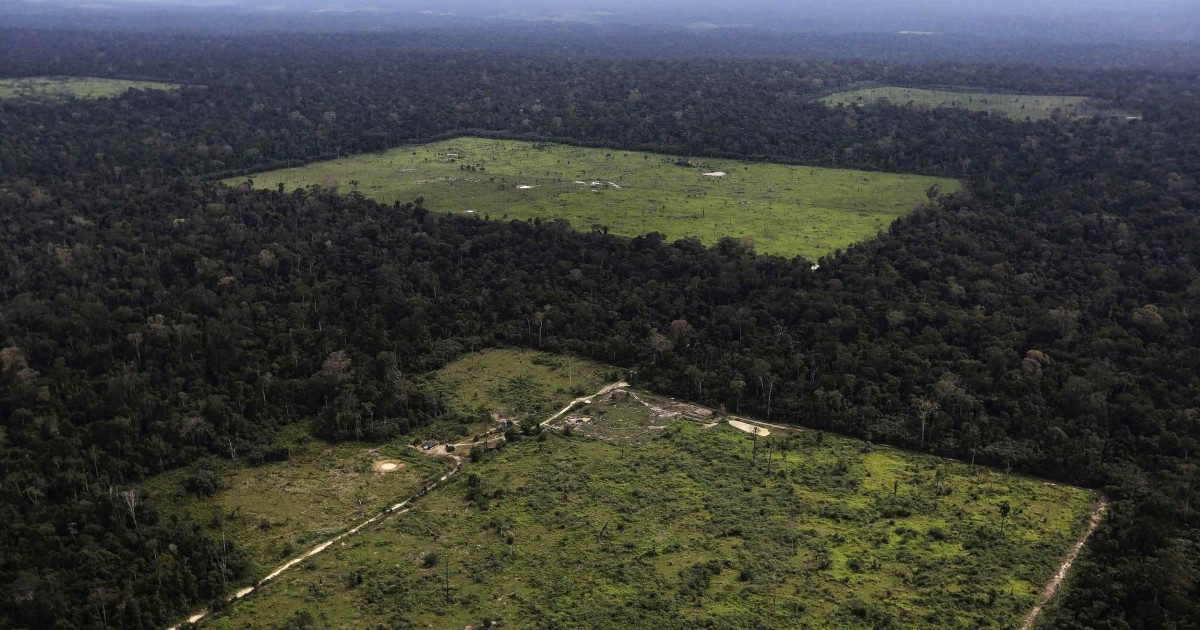This aerial, photorealistic landscape photograph captures a tropical rainforest scene with dense, dark green foliage, interrupted by four rectangular patches of cleared fields spaced hundreds of feet apart. The fields, likely intended for grazing, feature light lime green grass in stark contrast to the surrounding forest. A dirt road meanders through the lower portion of the image, where a few buildings are visible. The clearing nearest to the viewer, seen from a bird's eye perspective, contains some man-made structures that could be pipes or oil drilling machinery. The image is slightly foggy, adding to the depth and realism of the scene.